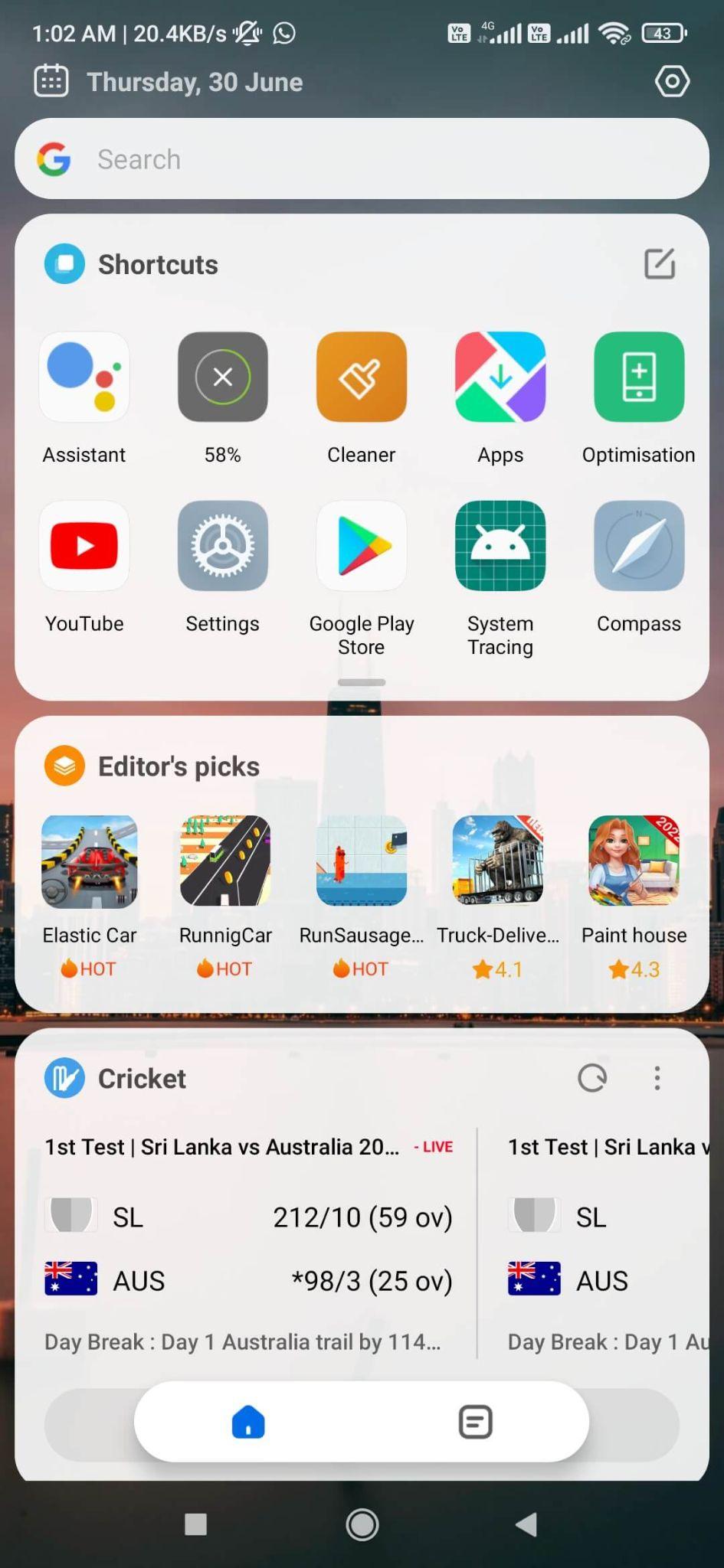A detailed screenshot of a smartphone display highlights an active website on the screen. At the top, there is a time display reading "1:02 a.m." along with the date "Thursday, 30th of June," preceded by a small calendar icon. Below this is the familiar Google search bar. 

A rectangular section labeled "Shortcuts" features a blue circle with a white square icon. Within this section are two rows of icons, each row containing five icons:

1. **Assistant**: A white square displaying a blue circle, a small red circle, and a tiny yellow circle.
2. **Battery Status**: A black square with a white circle outline and an 'X' inside, showing "58%".
3. **Cleaner**: An orange square with a white broom icon.
4. **Apps**: A colorful square with sections in red, blue, purple, and green, including a green downward arrow.
5. **Optimization**: A green square enclosing a white square with a plus sign.
6. **YouTube**: A red rectangle with a white play button inside.
7. **Settings**: A gray square featuring a gear resembling a steering wheel.
8. **Google Play Store**: A multicolored triangle in blue, green, yellow, and red.
9. **System Tracking**: A green button with white vertical and horizontal lines, forming a minimalist robot face.
10. **Compass**: A gray square with a compass icon inside.

Below the "Shortcuts" section is an "Editor's Pick" segment showcasing five game icons:

1. **Elastic Car**
2. **Running Car**
3. **Run Sausage**
4. **Truck Delivery**
5. **Paint House**

Further down, there is a sports update displayed in a white rectangle titled "Cricket". It provides real-time information about the first test match between Sri Lanka and Australia. The section outlines:

- "First Test Sri Lanka vs Australia"
- A score comparison between "SL" and "Australia"
- Note that "Australia trail by 114"
- Additional details: "Day break Day 1 Australia," "1 test Sri Lanka," with team names and flags, and an encapsulated segment with icons, including a blue house on the left and a black page-like symbol on the right.

The detailed layout and various icons within this screenshot collectively reflect a typical, content-rich smartphone interface.